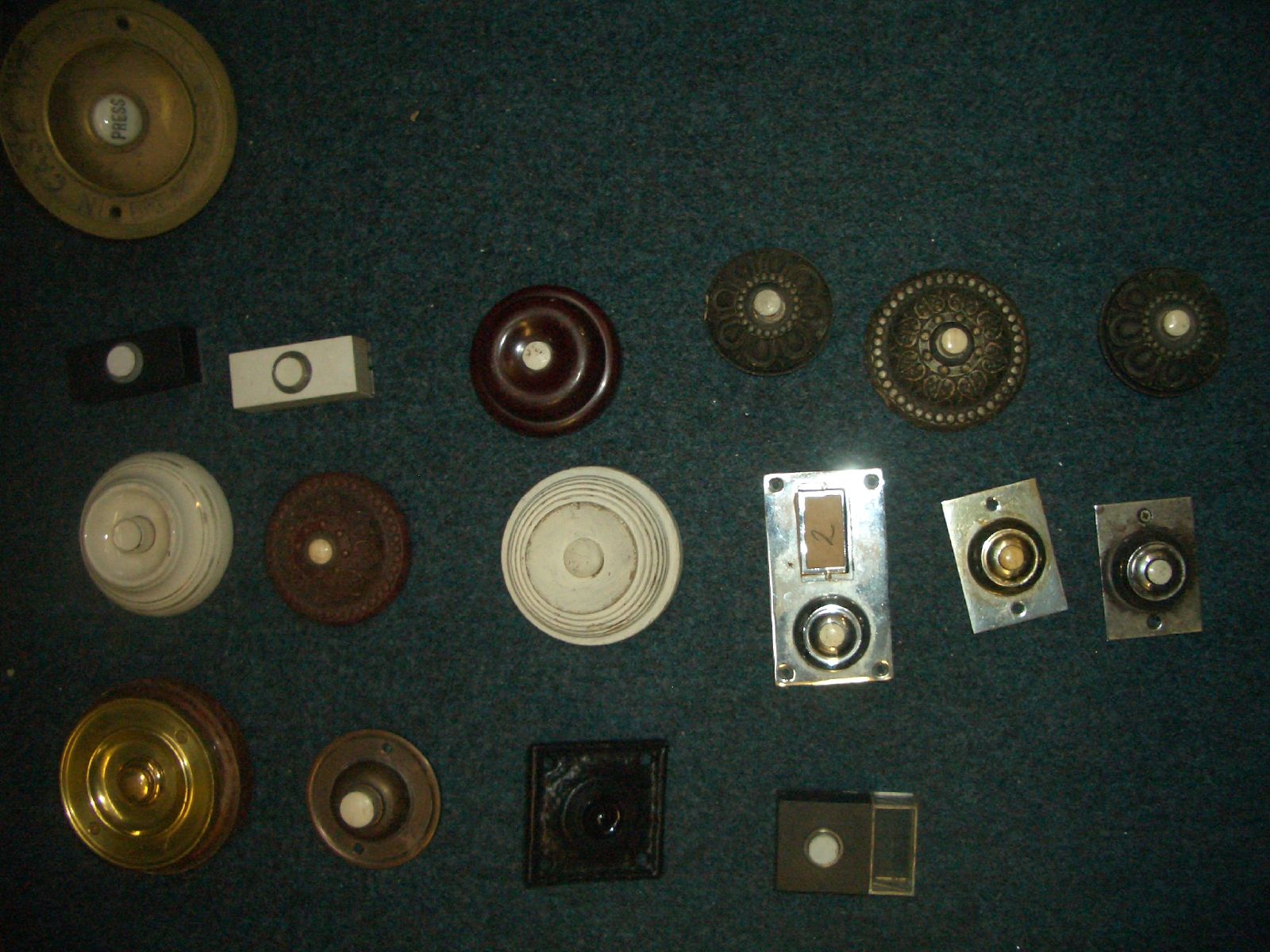A visually striking assortment of vintage doorbells is meticulously arranged against a dark blue backdrop. In the top left corner, a prominent, round brass doorbell stands out, featuring a central button inscribed with "PRESS." Below it, two rectangular doorbells are aligned—one is black and the other white, both with central white buttons. Adjacent to these, there is a round brown doorbell with a white button. A series of three sleek metallic doorbells with white buttons follow. 

On the next row, there's a white doorbell with a white button, a brown doorbell with a white button, and another similar white one. A long rectangular metallic doorbell marked with the number "2" has a white button at its base. This row is completed by two short rectangular metallic doorbells with central white buttons. 

The bottom row starts with a brown and gold doorbell featuring a gold button, followed by a brown doorbell with a white button, a black doorbell sans button, and a uniquely shaped sideways rectangular doorbell characterized by a black square and a central white button. Despite their varied designs and colors, these vintage doorbells share a common feature: a centrally placed button. The image is further distinguished by an underlying green carpet, enhancing the intriguing, almost surreal quality of this eclectic collection.